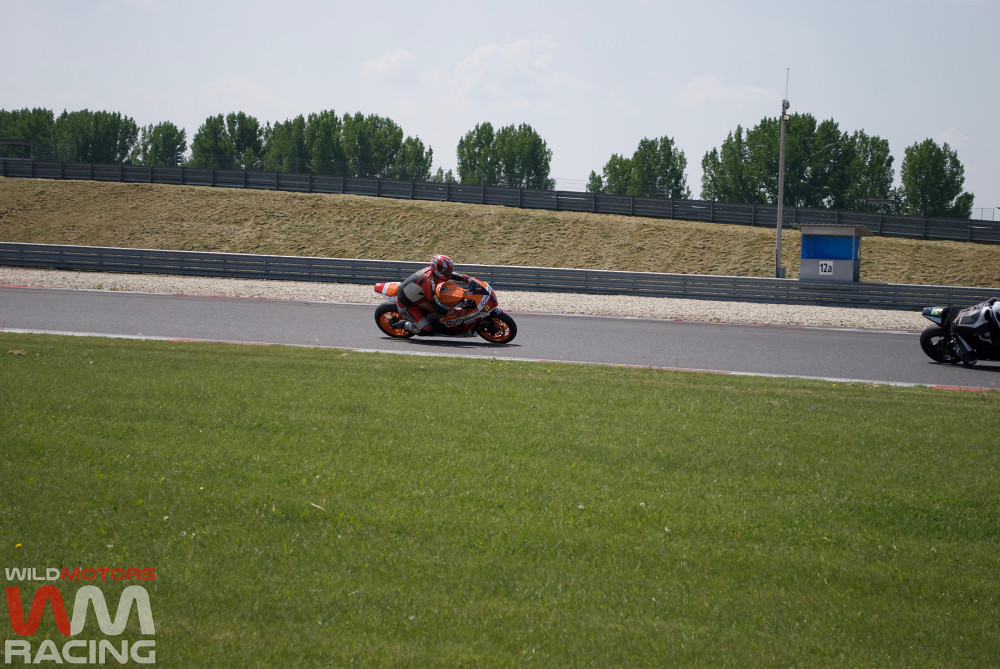In this detailed image of a motorcycle race set on a closed professional racetrack, a motorcyclist dressed in an orange and red outfit with a matching red and white helmet is captured executing a steep right turn on an orange and red motorcycle. Ahead of him, approximately 10 to 15 feet, the lower tail end and body of another motorcyclist clad in black can be seen, though the front half of their motorcycle is obscured. The riders navigate a narrow, unmarked concrete road set slightly back from the vantage point of the photographer. Dominating the image, a verdant green field stretches along the bottom half, leading into a distant backdrop featuring a fence and trees that delineate the track's boundary. The sky, dotted with clouds, suggests it is midday. Additionally, in the bottom left corner of the photograph, a logo reading "Wild Motors WM Racing" is prominently displayed. Further into the field, the marking "12A" is visible, reinforcing the competitive context of the scene. The array of colors in the photograph includes tan, orange, green, gray, white, brown, pink, and light blue, creating a vibrant outdoor setting.